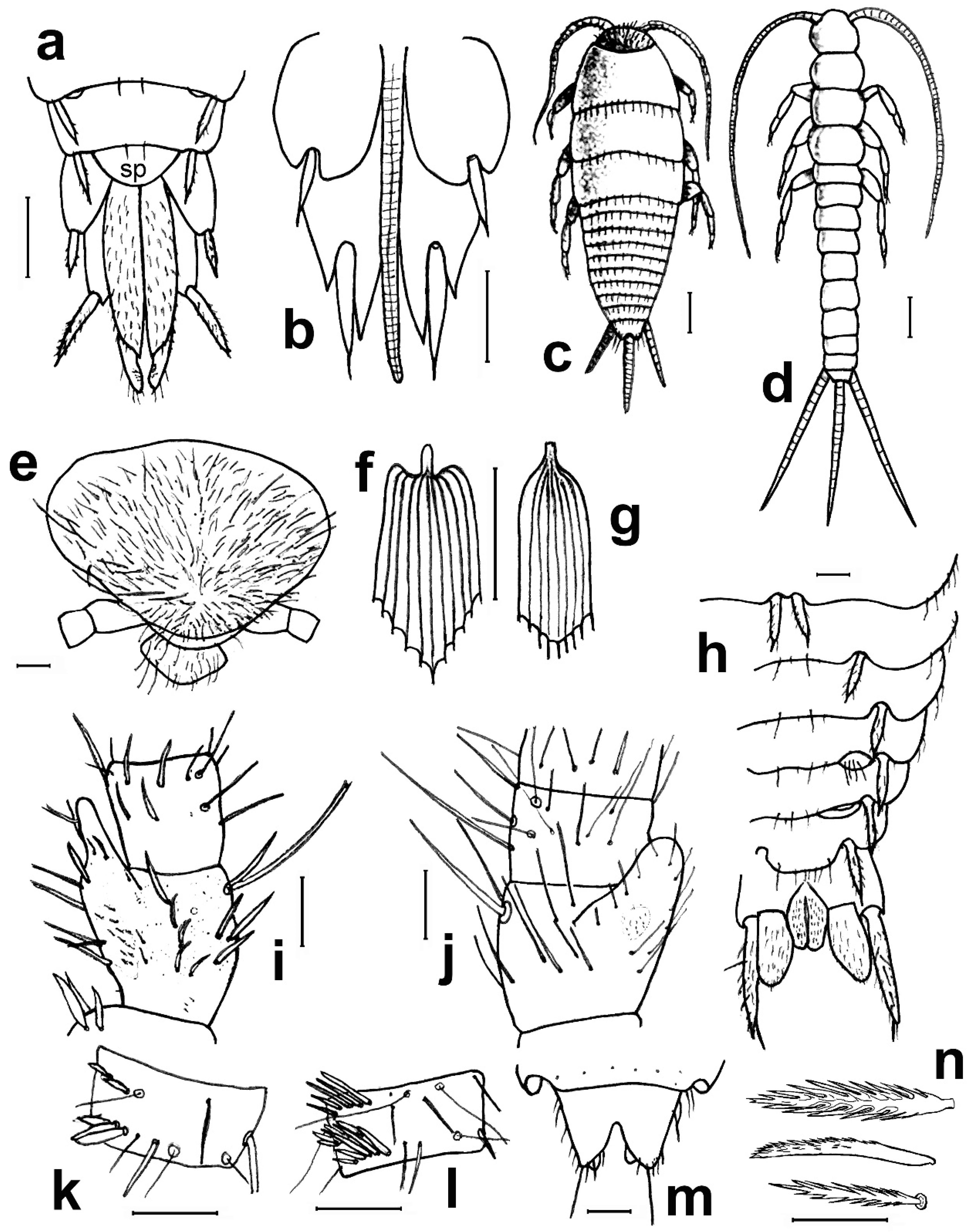The image is a detailed, black-and-white hand-drawn diagram, meticulously labeled from A to N, showcasing various parts of a certain insect, possibly a water bug or a similar creature. The diagram features enlarged views of the insect’s anatomy at a microscopic level, highlighting intricate details such as the shell, legs, mandibles, and even thorned and spined body sections. Larger, more comprehensive depictions of the insect are provided in sections C and D, illustrating the body and main carcass. The image serves as an informative poster to identify different parts of the insect, revealing features like six legs, large antennas, and hair-like whiskers, making it an educational yet eerie representation of the creature's anatomy.